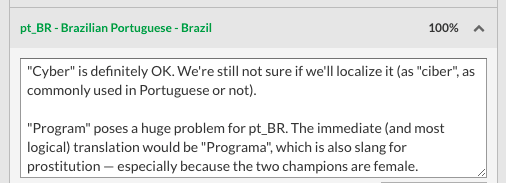This image features a white box within a gray border. At the top, green text reads "PT-BR (Brazilian Portuguese - Brazil)." Below this, bold text states "Cyber" (spelled "C-I-B-E-R") and mentions its acceptability while expressing uncertainty about its localization for the PT-BR market. Notably, "Cyber" can be used in Portuguese, but translating it as "programa" could pose issues. In Brazilian Portuguese, "programa" is slang for prostitution, which is particularly problematic because the context involves two female champions. The right side of the image contains the notation "100%."